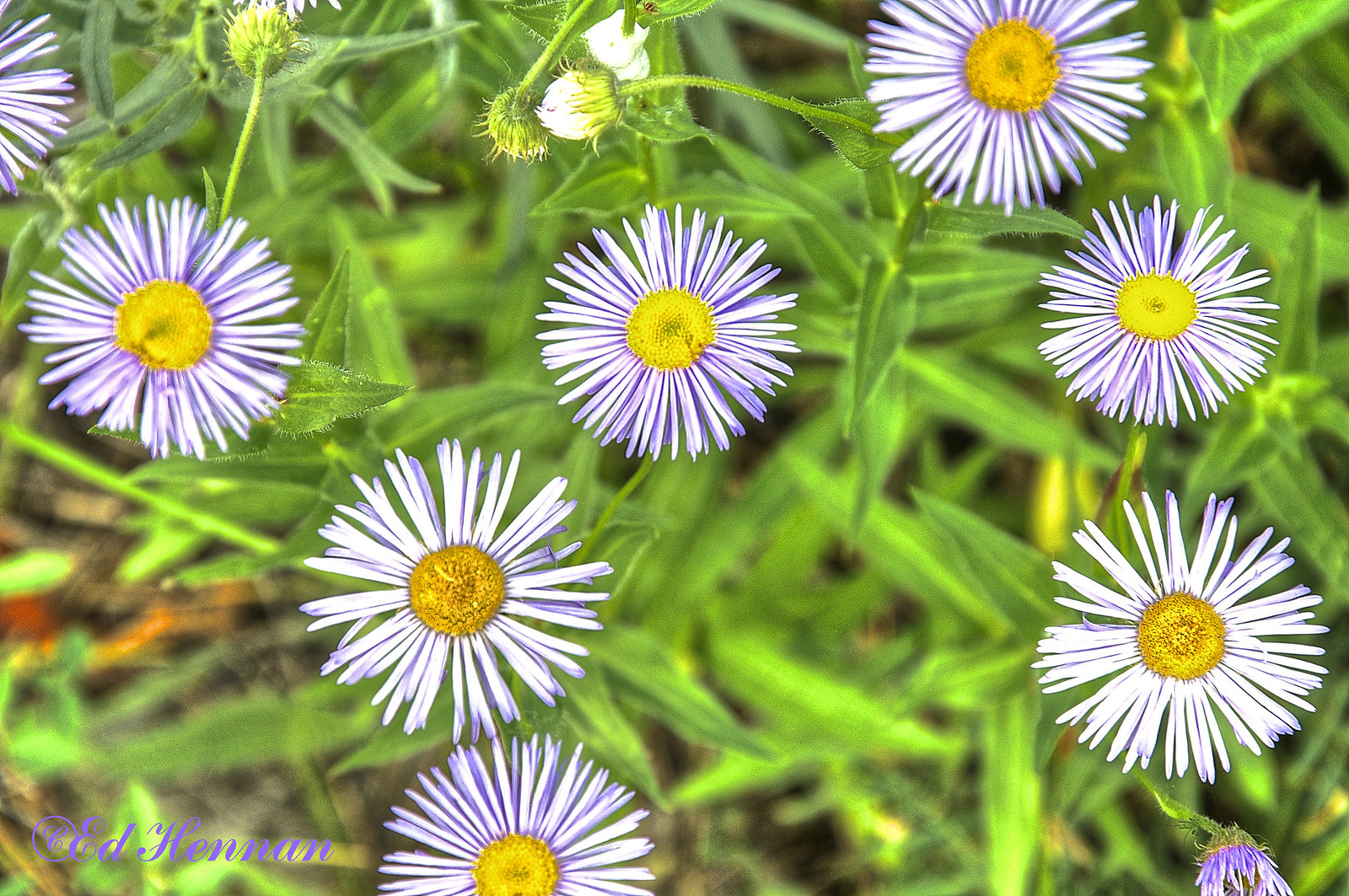The image is a very close-up photograph of several delicate flowers taken from a bird's-eye view. The flowers have incredibly thin, long petals that alternate shades of dark purple, light purple, and white, creating a striking contrast. At the center of each flower is a vibrant yellow core, rich with pollen. There are around six or seven flowers scattered throughout the image, along with four blooms that haven't yet opened near the top. The background is slightly blurry, showing hints of green leaves and possible brown shades that could be dirt. The picture has likely been enhanced to make the colors more vivid. In the bottom left corner, there is cursive purple lettering that reads "Ed Hinnon," or possibly "Ed Heernan."